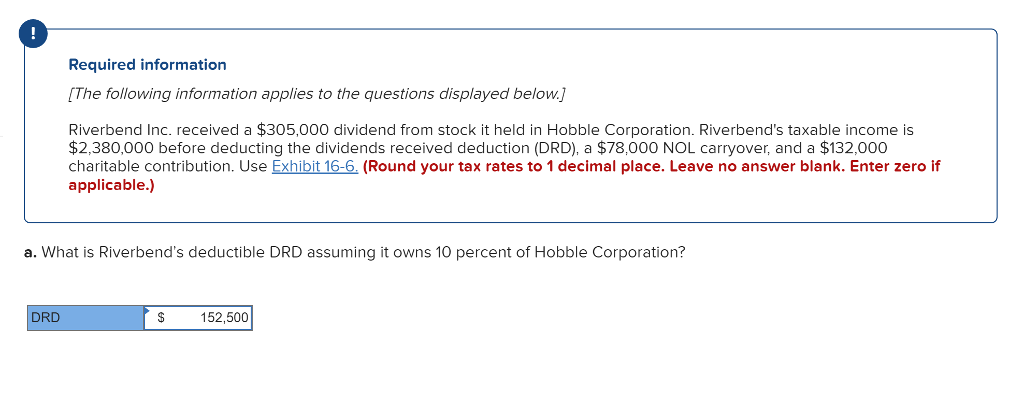The image is a screenshot presumably from a bank or investment account interface. The visible portion includes a notification box marked by an exclamation point in the top left corner. The alert, titled "Required Information," details the necessary data for the questions below. It specifies that Riverbend Inc. has received a $305,000 dividend from its stock in Hobby Corporation. Riverbend's taxable income, calculated prior to applying the Dividends Received Deduction (DRD), is $2,380,000. Additionally, Riverbend has a $78,000 Net Operating Loss (NOL) carryover and a $132,000 charitable contribution.

The notice advises users to refer to Exhibit 16-6 through a provided hyperlink and emphasizes in red text to round tax rates to one decimal place, ensure no answers are left blank, and to enter zero where applicable.

Beneath this notice is a question labeled "letter A," asking for Riverbend's deductible DRD, assuming it owns 10% of Hobby Corporation. In the answer box below, the calculated DRD is displayed as $152,500.

This seems to be a segment of a financial or taxation examination, requiring detailed numerical responses.